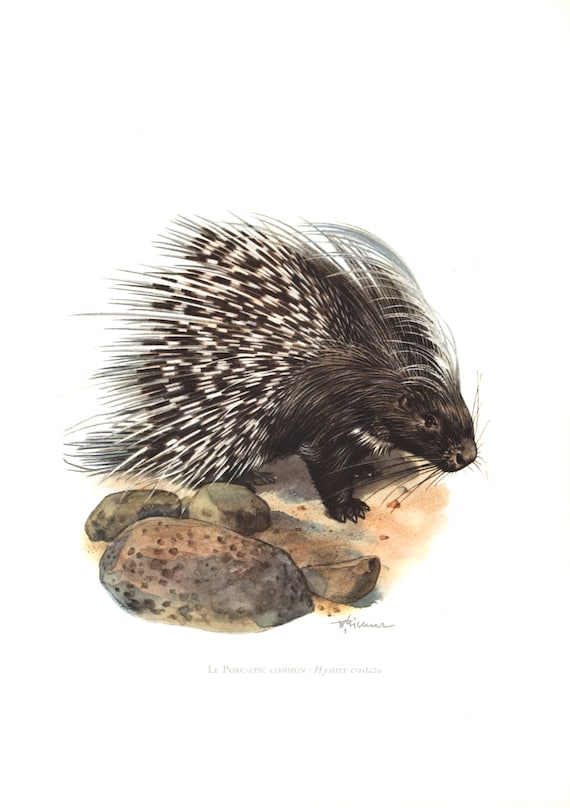The image is an illustration of a porcupine against a white background, rendered in a detailed watercolor style. The porcupine, facing to the right, is depicted primarily in black, with quills in varying hues of brown, white, and gray, creating a dynamic, multi-tonal effect. The quills give an impression almost like a mohawk of gray hair. Long whiskers extend from its nose, adding to the intricate detail of the drawing. The porcupine stands on a beige to cream-colored ground that resembles dirt or sand, with four small rocks scattered in front. At the bottom of the image, the artist's signature and the title "le porcupine" can be faintly seen inscribed in a very small gray font.